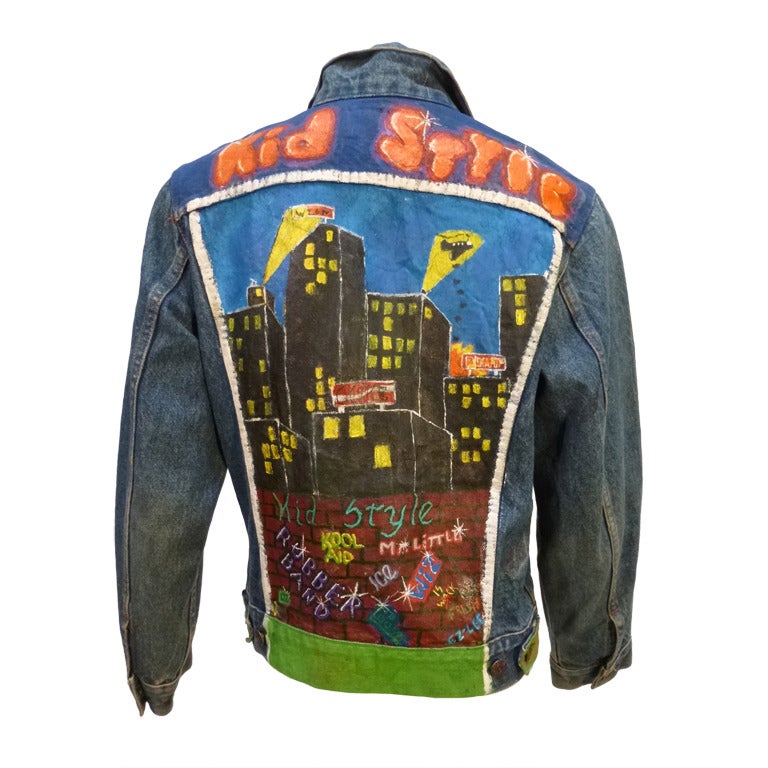This image is of a detailed, vintage-style denim jacket showcased on a white background, with the wearer edited out to focus solely on the jacket. The jacket features an ornate painting on the back, using what appears to be water-resistant paint. At the top, "Kid Style" is boldly inscribed in orange letters. Below this, a busy cityscape is depicted with tall black skyscrapers adorned with yellow-lit windows, set against a blue sky. Notably, yellow triangular kites are visible in the sky, adding a whimsical touch. A green horizontal stripe separates the upper section from a red brick wall at the bottom, which is scribbled with various graffiti phrases like "Kid Style," "Kool-Aid," "rubber bands," and "ice," evoking an urban, street-art aesthetic. The jacket's back design, with a white-bordered rectangle encompassing these vivid elements, gives it a unique and trendy flair suitable for a kid's stylish wardrobe.